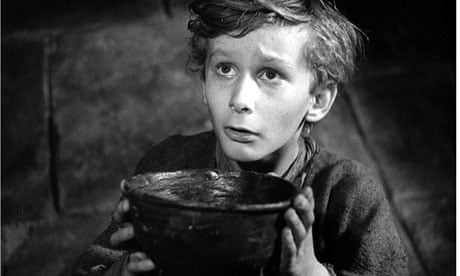This evocative black-and-white photograph, reminiscent of an old movie scene from the 1930s to the 1950s, captures a young, pale-skinned Caucasian boy directly in the center of the image. The boy, who appears to be dressed in tattered clothing and possibly homeless, kneels on a floor that resembles stone tile, holding up a small, black, empty bowl with both hands outstretched. His longer hair and worried, pleading eyes, along with his slightly open mouth, give him a desperate expression as if silently begging for food. The stark background, a darker charcoal gray that fades into a blur, adds to the poignant, grayscale composition, emphasizing the boy’s dire situation in this striking, cinematic portrayal.